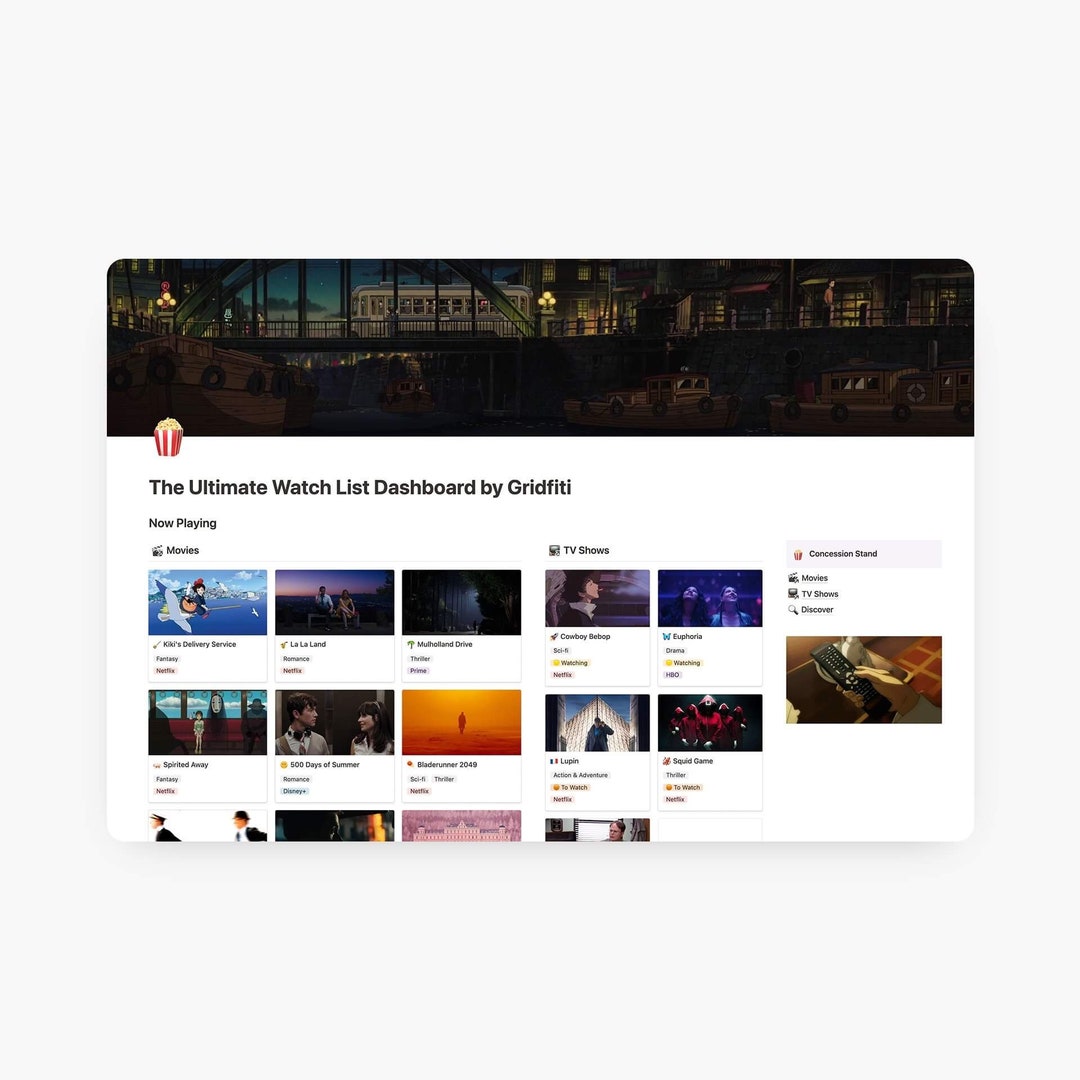This vertical image features a clean, medium gray background devoid of any texture or dimension. Centrally placed on this flat backdrop is a rounded-edge, horizontal dashboard designed for accessibility on computers and smart devices. 

At the top of the dashboard, there is a nighttime-themed image, perhaps suggestive of a movie atmosphere, accompanied by a small popcorn icon on the left-hand side. Bold black text below this image reads, "The Ultimate Watch List Dashboard by Gridfiti," followed by the phrase "Now Playing."

The dashboard is segmented into sections, one for movies and another for TV shows. Under the "Now Playing" movie section, a list of titles is presented along with their respective icons, genres, and streaming platforms. The movies displayed include:
- Kiki's Delivery Service
- La La Land
- Mulholland Drive
- Spirited Away
- 500 Days of Summer
- Blade Runner 2049

Three additional movie titles are partially shown at the bottom of the list. Each movie entry includes a thumbnail image, the title, the genre (such as fantasy or romance), and the platform where it is available for streaming (like Netflix, Prime, or Disney Plus).

The TV shows section follows a similar format, listing the show titles along with their icons, genres, and streaming platforms. Notable TV shows listed include:
- Cowboy Bebop
- Euphoria
- Squid Game

One more TV show title is partially visible at the bottom of this section.

Additionally, a concession stand icon featuring popcorn is displayed, alongside options labeled "Movies," "TV Shows," and "Discover." The image captures the essence of streaming convenience with a person shown clicking a remote.